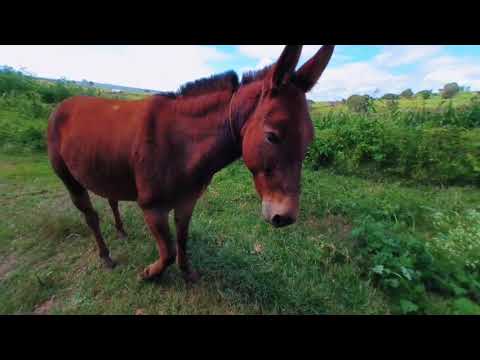A reddish-skinned donkey, with black spiky hair, stands in a grassy field under a blue sky filled with white clouds. The grass around him is very green, suggesting it might be spring or summer, and it is low to the ground, possibly from grazing. He is positioned at an angle to the camera, allowing a full view of his body length. His head is perpendicular to the ground, and he lifts his right leg, as if in mid-step. There is no harness or bridle on him, indicating he is not a riding animal. The field is slightly weedy on the right side. Gentle, undramatic hills roll in the background. Black bars frame the top and bottom of the image, giving it a cinematic feel.